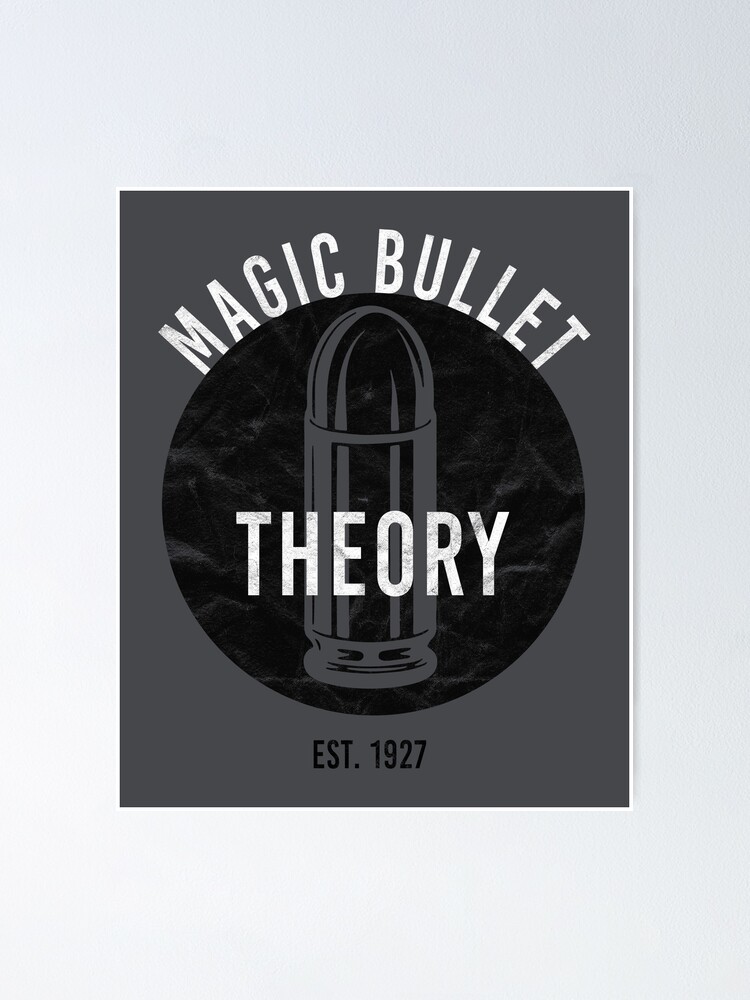The image is predominantly grayscale, featuring a poster-like design set against a gray background. At the center of the image is a dark gray rectangle, which houses a prominent black circle. Inside this circle, there is a gray outline of a standing bullet, detailed with grooves and markings. Overlaid on the bullet are the words "Magic Bullet Theory" in bold white text. Just beneath this, in smaller black lettering, it reads "EST 1927." The overall design is minimalist, using a combination of black, white, and various shades of gray to create a striking, focused composition with the bullet as the central element.